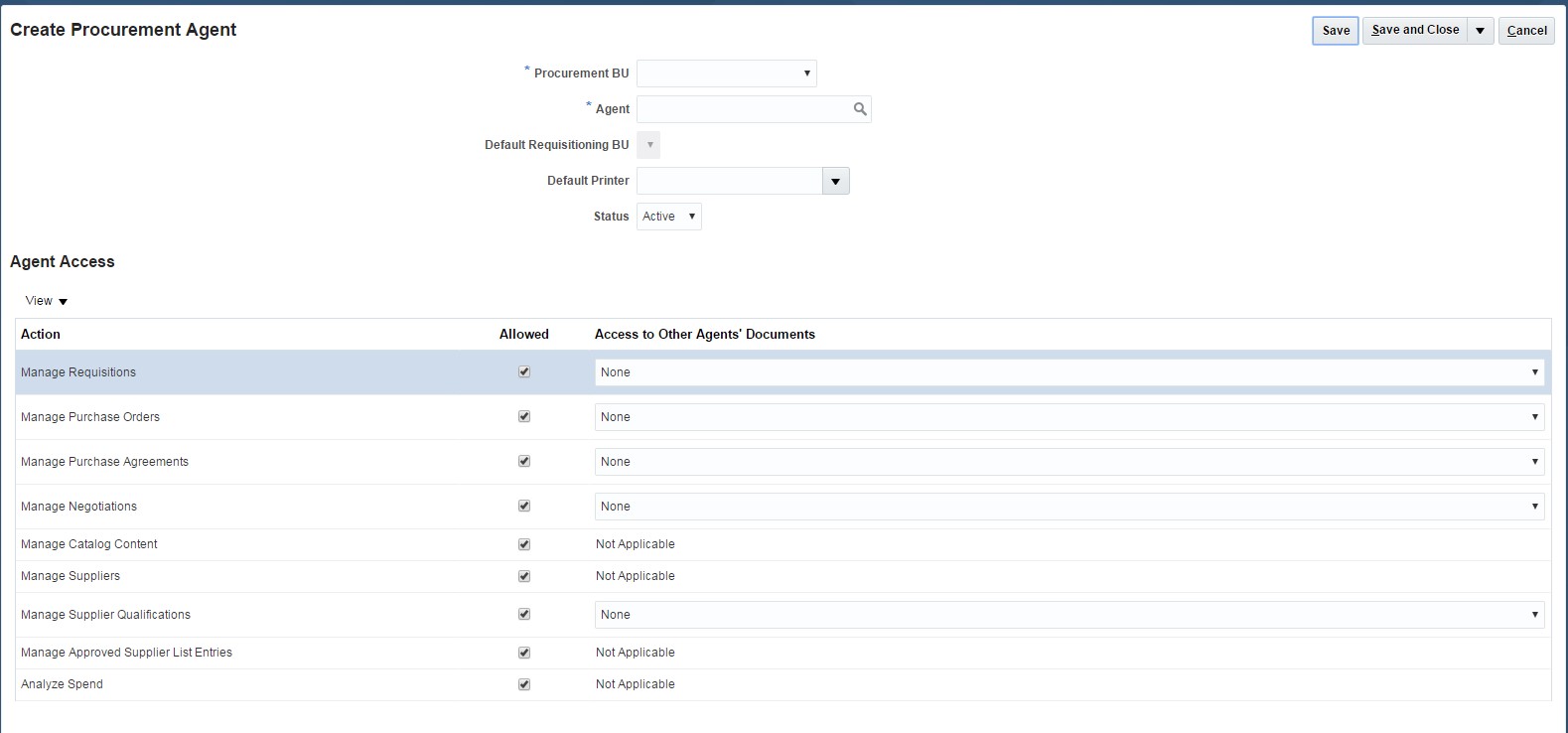On the left side of the image, "Create Procurement Agent" is written in black text. On the far right, inside a blue square, the word "Save" is displayed. Next to it, there are two more options: "Save and Close" and "Cancel" inside a gray square.

The options in the interface begin with the label "Agent" followed by a search bar with a magnifying glass icon. Below that, the word "Default" is accompanied by another search bar. Next is "Default Premier" with yet another search bar area, an arrow pointing down, and the word "Status" beside it, indicating "Active".

Beneath this section, the heading "Agent Access" is followed by the word "Action". Below this, there is a long blue rectangle that states "Manage Requesters" with the word "Allowed" displayed to the right. Directly underneath "Allowed," there is a checkbox.

The next category header in black text reads "Access to Other Agents' Documents." Within this section, there is a search box containing the word "None."

Returning to the "Agent Access" section, the option "Manage Purchase Orders" is displayed along with a checked box. Similarly, the label "None" appears underneath "Access to Other Agents' Documents."